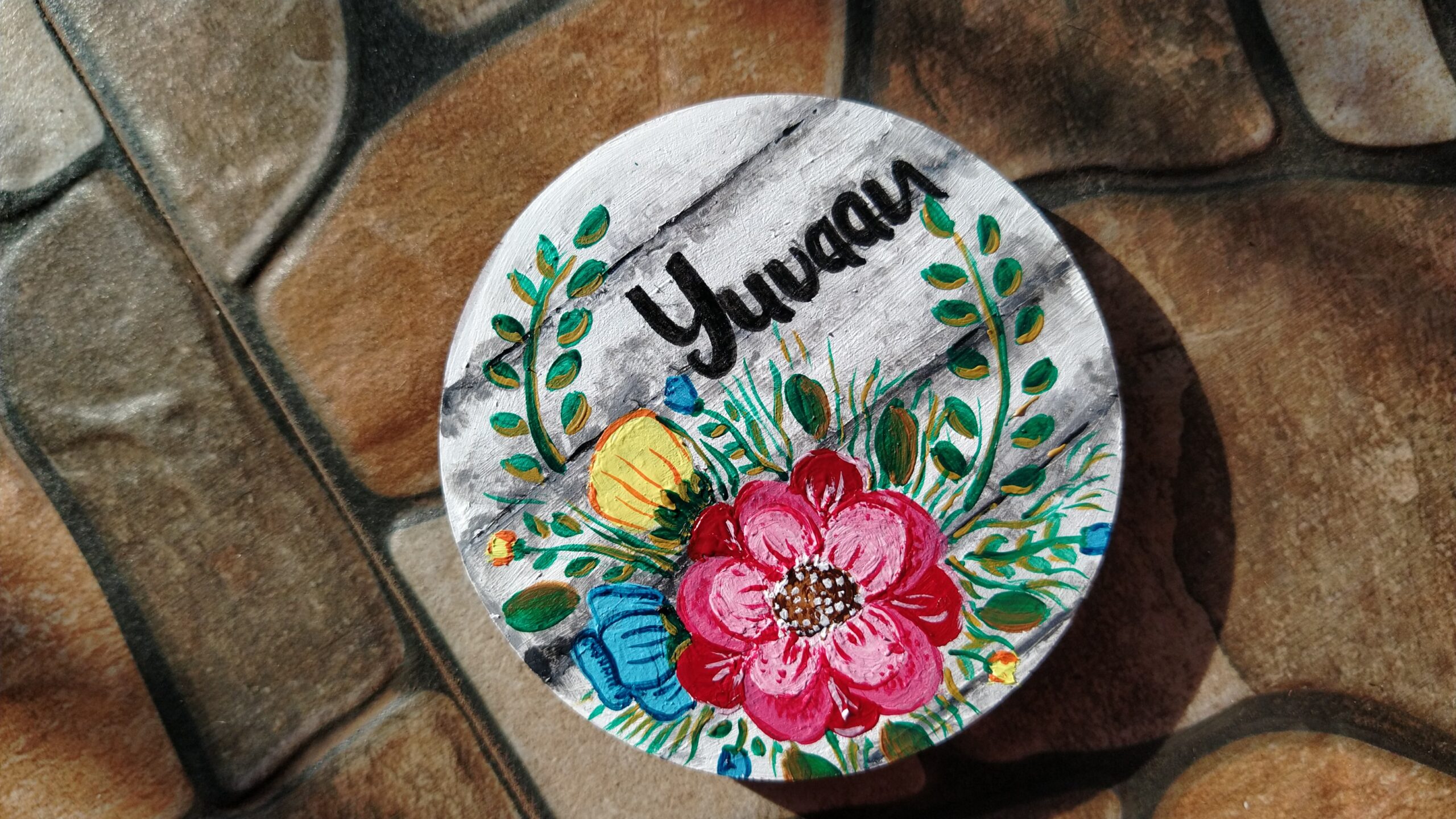The image depicts a circular decorative plate resting on a surface of artificial stone pavers in various shades of tan and gray. The plate features a detailed and vibrant painting of a bouquet of flowers. This bouquet includes one prominent red and pink flower in the foreground, two yellow flowers—one large and one very tiny—in the background, and a blue flower. The white background of the plate is accented with gray lines, enhancing the design. Additionally, green and yellow leaves extend around the edges of the painted flowers. The plate, which has a high-quality finish, also displays a text in bold black letters that reads "Y-U-U-A-A-N," with the 'N' appearing backwards.